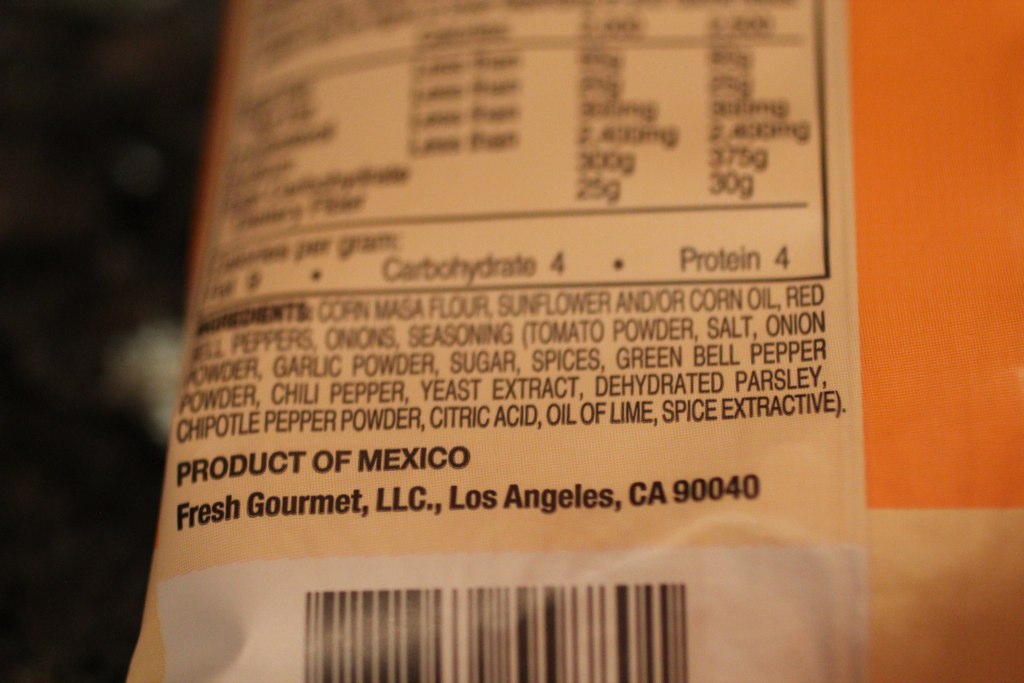This detailed close-up image captures the ingredient label on the back of a partially visible orange food package, likely made of plastic. The prominent text on the white label with black text reads "Product of Mexico, Fresh Gourmet, LLC, Los Angeles, California, 90040," with a barcode below. The main ingredients listed are corn, masa flour, sunflower and/or corn oil, red and green bell peppers, onions, tomato powder, salt, onion powder, garlic powder, sugar, spices, green bell pepper powder, chili pepper, yeast extract, dehydrated parsley, chipotle pepper powder, citric acid, and oil of lime. The picture also displays partial nutritional information, noting four grams of carbohydrates and four grams of protein, though the rest of the nutritional chart is blurry. The label and ingredients are sharp and clear, while the rest of the package and background are out of focus, emphasizing the detailed ingredient information.